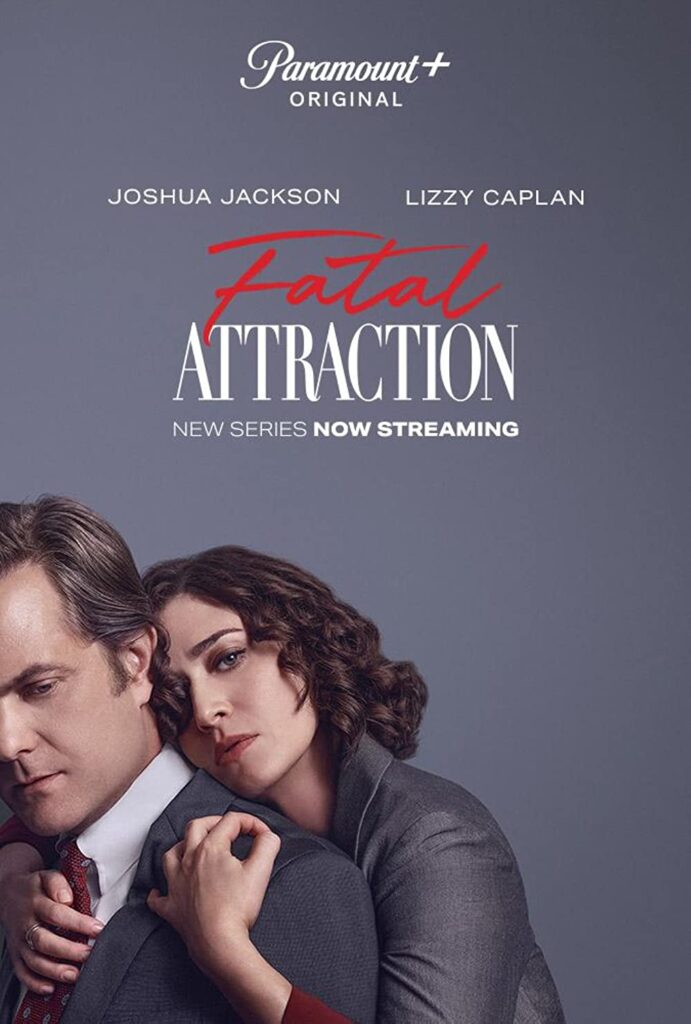This poster advertises a TV show with a gray background. At the top, "Paramount Plus Original" is written in white Paramount font. Below that, the names "Joshua Jackson" and "Lizzie Kaplan" are in plain white font. Prominently in the center, "Fatal" is written in large red letters, followed by "Attraction" in large white font. Underneath, "A New Series Now Streaming" is also in white. At the bottom, the two actors, Joshua Jackson and Lizzie Kaplan, appear. Joshua Jackson, a white man with dark hair, is dressed in a gray suit and white shirt, looking down pensively. Behind him, Lizzie Kaplan, with dark hair, chiseled features, dark eyebrows, and brownish lipstick, wears a gray jacket and clutches him from behind, staring intensely at the camera.